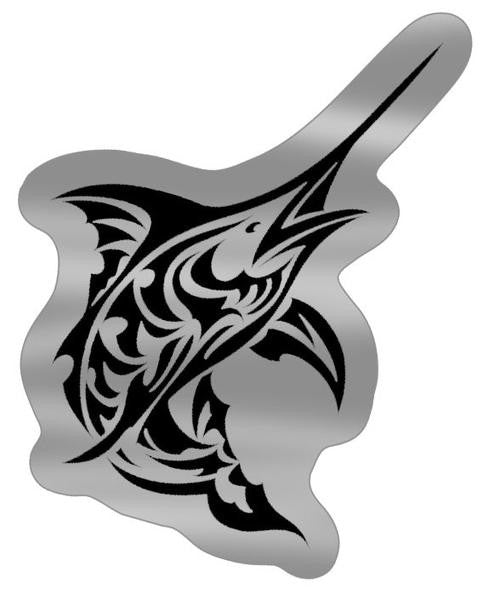This image features an intricately designed swordfish, rendered in black with silver highlights, and framed by a metallic silver cutout that suggests it could be a sticker or a metal token. The swordfish is artfully depicted with paisley-like silver swirls and elaborate curves, giving it a tattoo-like aesthetic. Twisting elegantly from the middle of its torso to its tail, the fish's extended sword points up and to the right. Both the large, expansive tail and the sharp fins are adorned with detailed accents, and the fish's slightly open mouth adds a touch of realism to the otherwise artistic portrayal. The balanced silver border surrounding the black and silver swordfish completes the design, enhancing its overall visual impact.